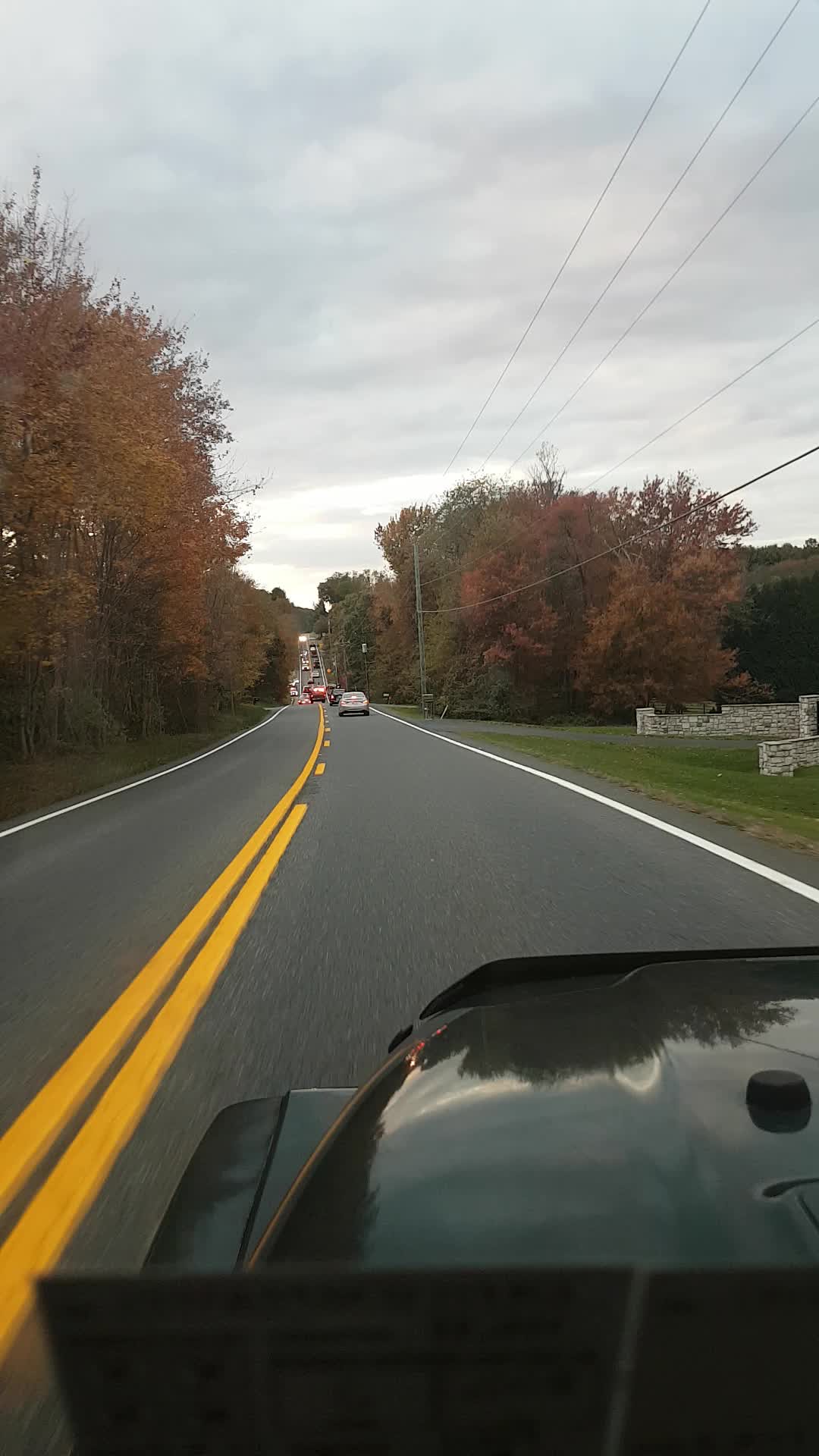This image, captured from a dash cam in a gray SUV, shows a busy country road lined with autumnal trees displaying vibrant fall foliage in shades of gold and red. The road appears newly paved and is situated in a wooded area with gray clouds overhead, suggesting an overcast fall day. Electric wires run parallel to the road on wooden poles. To the right, there is a large, grand entryway made of white stone, possibly leading to a house or subdivision. The road features two yellow lines marking the center and a solid white line on the right. A line of cars stretches ahead, leading up to an intersection in the distance, from which several cars are approaching. The overall scene conveys the busyness of the road despite its rural setting, enhanced by the beautiful fall colors enveloping the area.